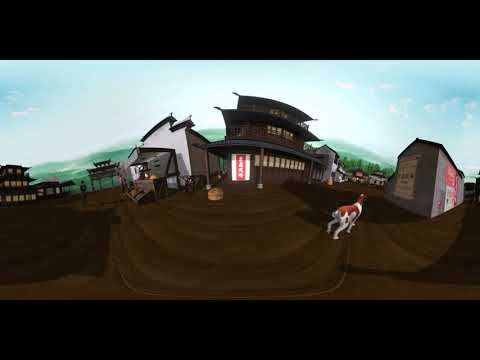This is an animated image depicting a western-style town. At the center is a large, brown, pagoda-like saloon with three tiers and numerous windows on each floor. To the left of the saloon is a white building with brown trim, which features a food stand on its side. On the right side of the image, there is a smaller, gray building adorned with various signs, resembling a barn. The entire scene is set on dirt hill-like ground. In the foreground stands a small, white dog with brown spots, gazing towards the gray building. The background showcases rolling green hills beneath a bright blue sky with some white clouds. The image is highly digitized, giving it a computerized appearance typical of a video game screenshot.